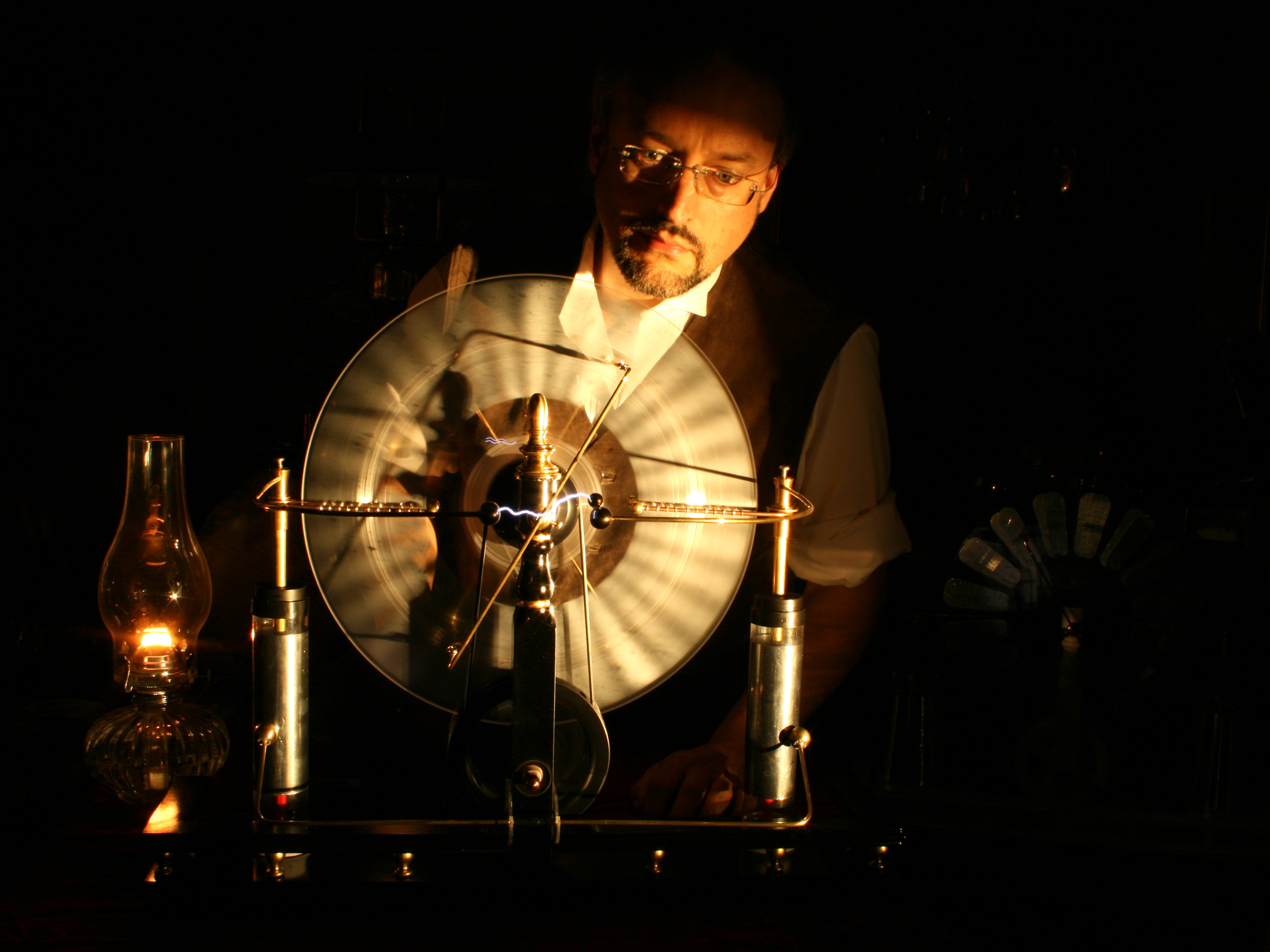The image captures a detailed scene of a middle-aged white man, sporting glasses, a mustache, and a goatee, gazing intently downward. He is inside a dimly lit room, wearing a white shirt with rolled-up sleeves and a dark vest. The focal point in front of him is a complex contraption. At the center of this apparatus is a fan-like structure with blades in motion. Flanking the fan on both sides are two silver metal cylinders connected by wires, with electrical currents visibly sparking between them. To the left of this setup is a burning oil or gas lamp, contributing to the overall dark ambiance of the setting. Various indistinct objects and shadows are present in the background, adding to the mysterious and scientific atmosphere of the scene. This photographic image captures the man deeply engaged in what appears to be a scientific experiment, immersed in his work.